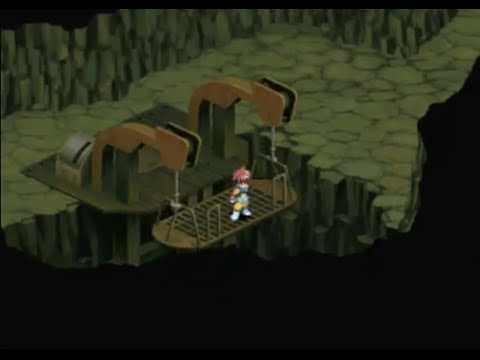In this screen grab from a video game, a character with pink hair, dark sunglasses, a yellow shirt, and white boots stands on a metal platform suspended by two overhead brown cranes. The platform, appearing to be part of a pulley system, hangs over a dark abyss against a primarily black background. The scene features a rocky formation, resembling a stone-covered walkway with a large, steep rock formation towering behind it. The environment suggests a mining or mountainous area, with green cliffs and upright green pillars forming the background. The image lacks any text, interface, control panels, or menus, presenting a clean, focused depiction of the character poised to be lowered into the abyss below.